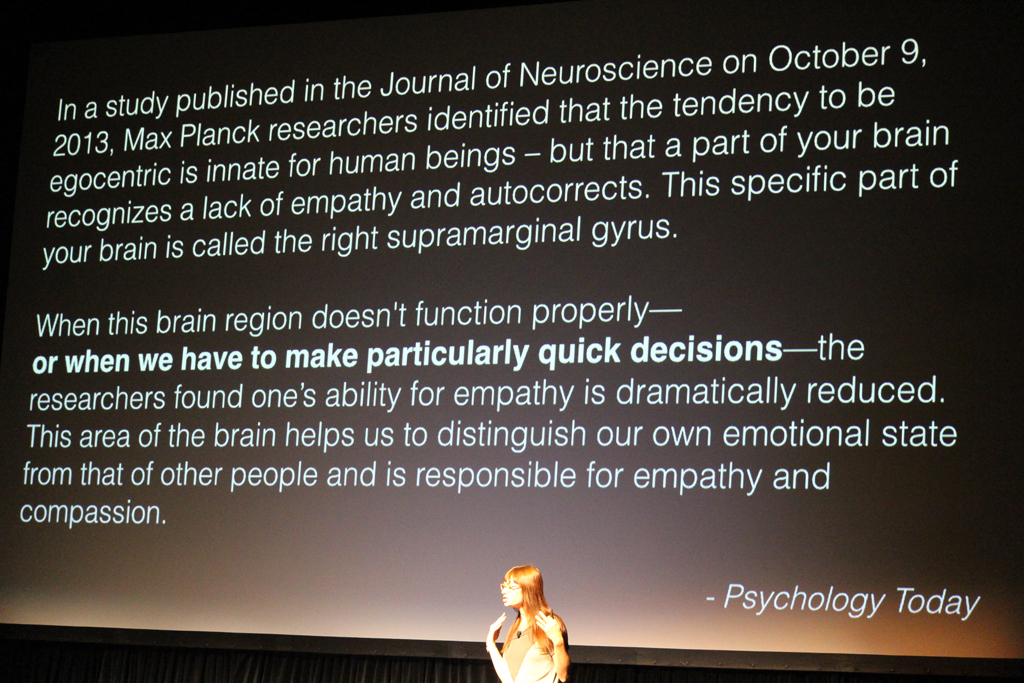In the photograph, a young woman with long red hair and glasses stands to the left of a large projection screen, facing towards it while gesticulating animatedly with both hands, as if explaining or giving a lecture. She has a microphone clipped to her collar, further suggesting she is presenting to an audience. The projection behind her features a gradation background transitioning from dark to lighter brown, with two paragraphs of white text. The text begins, "In a study published in the Journal of Neuroscience on October 9, 2013, Max Planck researchers identified that a tendency to be egocentric is innate for human beings, but that a major part of your brain recognizes a lack of empathy and autocorrects. This specific part of your brain is called the right supramarginal gyrus." The second paragraph states, "When this brain region doesn't function properly or when we have to make particularly quick decisions, the researchers found one's ability for empathy is dramatically reduced. This area of the brain helps us distinguish our own emotional state from that of other people and is responsible for empathy and compassion." The credit "Psychology Today" is noted in the bottom right corner of the screen.